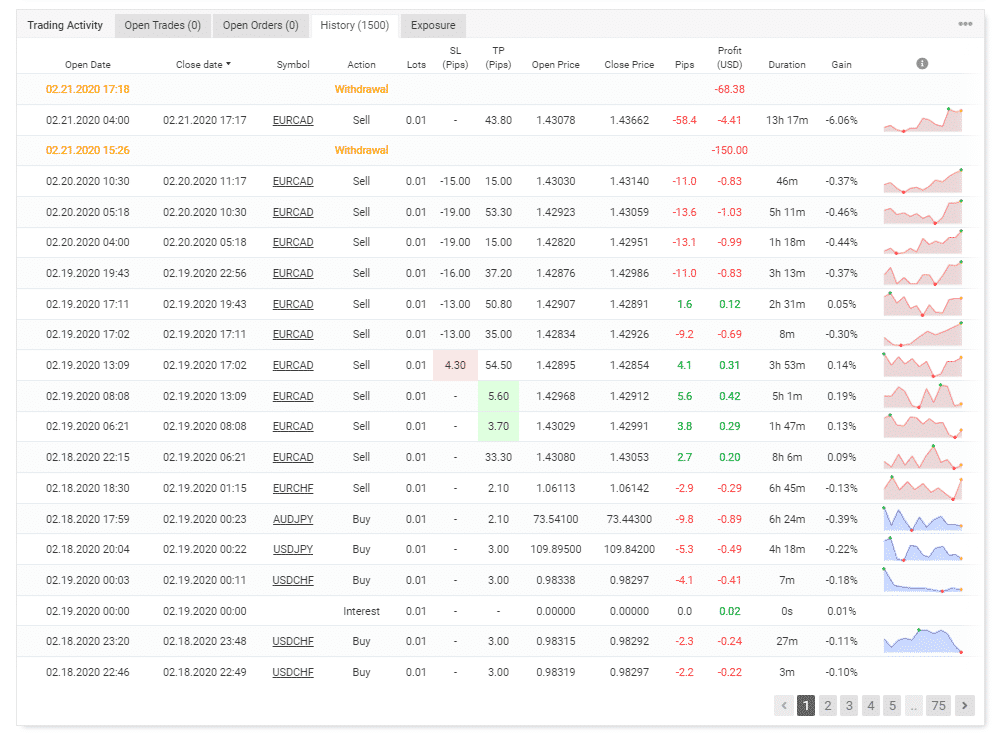The webpage currently being viewed is dedicated to forex trading or currency exchange, specifically designed for individuals with private trading accounts. The interface features multiple tabs at the top: "Trading Activity," "Open Trades" (indicating zero open trades), "Open Orders" (also showing zero open orders), "History" (documenting over 1500 trades), and "Exposure."

Below the tabs, there is an organized list featuring detailed information for each trade. The columns include the open date and close date of trades, the symbols representing the types of forex or currencies being exchanged, and the action or disposition associated with each trade. Further columns detail the number of lots traded, pips (price interest points), SLTP (Stop Loss and Take Profit), along with the open price and close price.

Additionally, there's a column for pips again, followed by the profit earned, which is displayed in USD. Here, negative values are shown in red, indicating losses, while positive values are highlighted in green, indicating gains. Other columns include the duration of each trade and the overall gain. At the far end of the page are small graphs in red and blue, visually illustrating the fluctuations and trends of the trades.